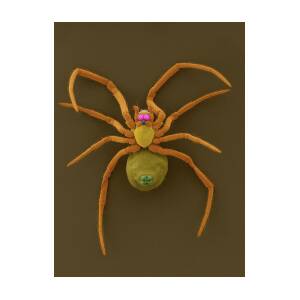The image depicts a lifelike, handcrafted spider made from felt and various craft materials, positioned on its back against a plain, dark brown background. The spider features eight fuzzy, light brown legs, each adorned with a hint of burnt orange. Four legs extend on each side, with the front pair slightly curled inward. The underside of its abdomen is striking green, reminiscent of a kiwi fruit's texture, complete with an emerald green dot at the tip where the spinnerets would be. Its thorax and head are tan, with an egg-shaped yellow shape in the center where all legs converge, possibly resembling an egg sac. The spider's head is accented with two unrealistic, glowing pink eyes, contributing to its surreal appearance. This meticulously crafted spider is about the size of an adult human hand and presents a photorealistic style, despite its evident artificiality.